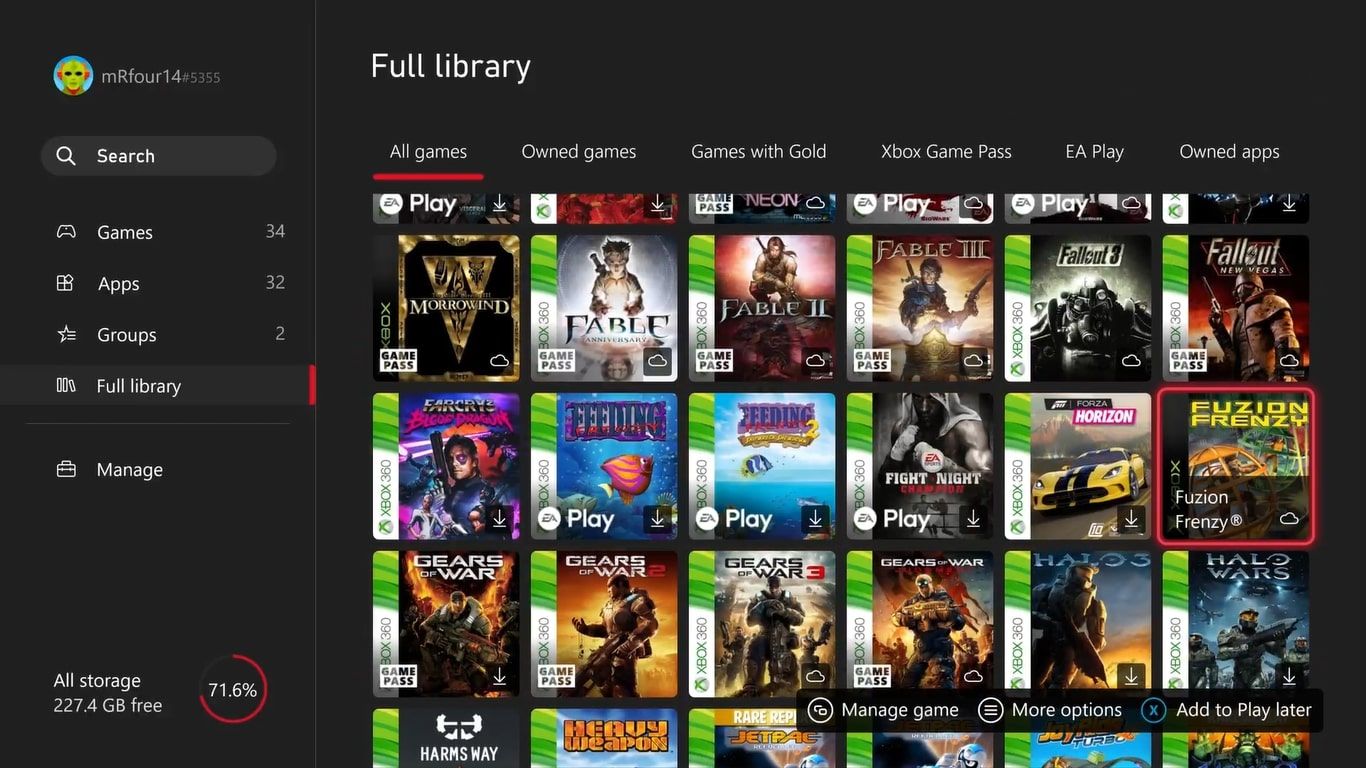Screenshot of the Games Library

The screenshot displays a detailed view of a user's games library interface. On the left side, there is a prominent sidebar with several elements:

- At the top, the user's name is displayed: "Mr414 #5355,” accompanied by a circular profile picture featuring an alien.
- Below the username is a pill-shaped search button for conveniently finding content.
- Underneath the search button, there are five specific buttons, each with an icon on the left side. These buttons are labeled:
  - Games (34)
  - Apps (32)
  - Groups (2)
  - Full Library
- At the bottom of the sidebar, there is storage information indicating 227.4 GB of free space accompanied by a circular progress bar showing 17.6% usage.

To the right of the sidebar, the main section of the screen displays the "Full Library" heading. Below this heading, six buttons are organized horizontally, each serving a categorization purpose:

- All Games (underlined in red to show it's currently selected)
- Owned Games
- Games with Gold
- Xbox 
- Game Pass
- EA Play

Beneath these buttons is a grid layout containing images of various games. There are six images in each row, but the top and bottom rows are partially cut off, leaving only the middle rows fully visible.